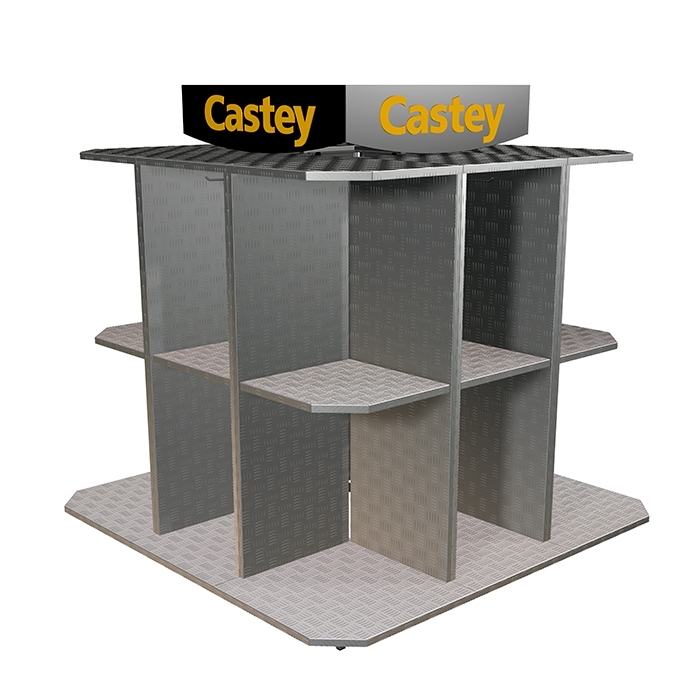The image features a metallic silver structure set against a white background. This structure appears to be a versatile, all-directional shelving unit with a square shape, constructed primarily from metal with a reinforced pattern that suggests recycled material, possibly resembling pieces of a truck bumper. It comprises three distinct horizontal metal plates—one on the top, one in the middle, and one at the bottom. The middle plate intersects four vertical metal sheets, creating a sturdy framework. The entire unit has an open design, making it accessible from all directions.

The shelving unit has two visible metal signs on top, positioned at an angle, with the brand name "Castey" prominently displayed in yellow letters. The sign on the left is black, while the one on the right is grey, both contributing to the distinctive brand identity atop the structure. The unit itself appears to be divided into multiple compartments or boxes, potentially offering various levels of storage within its square frame.